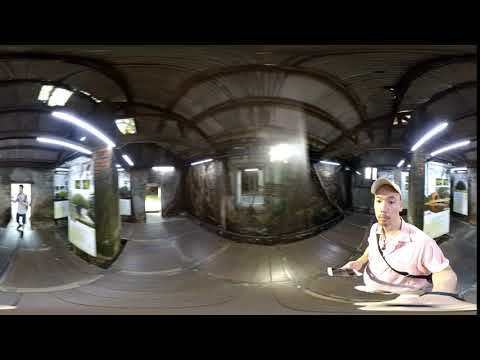The image features an Asian man with a mustache and a light pink collared shirt, buttoned down, and a white baseball cap. He's carrying a selfie stick with an outstretched arm, giving the impression he's taking the photo himself. The room around him appears distorted, creating an illusion that he's halfway submerged in the floor, though he's likely seated or standing. There is a strap running from his left shoulder to his right underarm, and in his other hand, he seems to hold a flashlight. 

The setting seems to be an old, slightly eerie building with dark brown, shiny metal walls and a curved ceiling. The floor is dark gray or brown. There are columns and multiple doors. One door on the left reveals someone standing in a white shirt and dark pants, possibly walking toward the camera. Another door in the background shows a couch with two hanging lights above it. The overall atmosphere is reminiscent of a cave-like or industrial space, with panoramic distortion adding to the surreal feel.